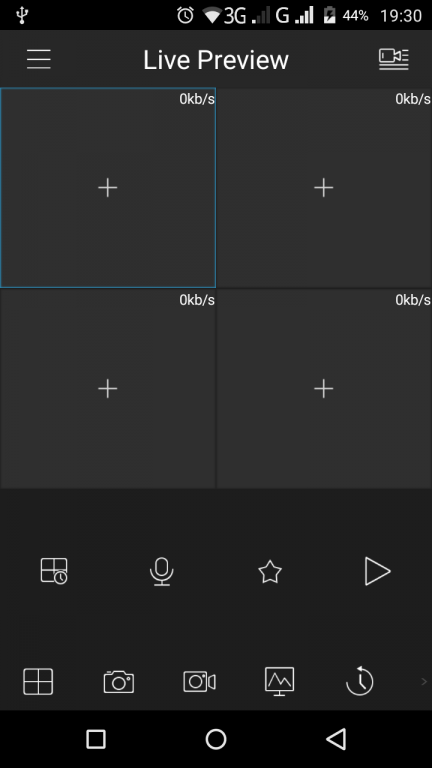This image is a screenshot of a mobile device displaying the interface of a video editing or broadcasting app with a black background. At the top of the screen, there is a horizontal menu with a list button on the left. In the middle, "Live Preview" is prominently displayed in white text, and to the right, there is an icon of a camera with lines extending in front and underneath it, symbolizing live recording or streaming.

Below the top menu, there are four square tiles aligned in a grid. Each tile has a white plus symbol in the center, suggesting that users can add content or footage to these slots. 

In the top right corner of the screen, there is a data usage indicator showing "0 kbps," indicating no data transfer or streaming activity at the moment.

The bottom portion of the screen is divided into two rows of icons. The first row includes icons resembling a tile with a timer, a microphone, a star, and a play button. The second row features another tile icon, a camera icon, a video camera icon, a usage or monitor icon, and finally, a timer icon.

Overall, the detailed functions and layout suggest a robust interface designed for managing video content, possibly for live broadcasting.